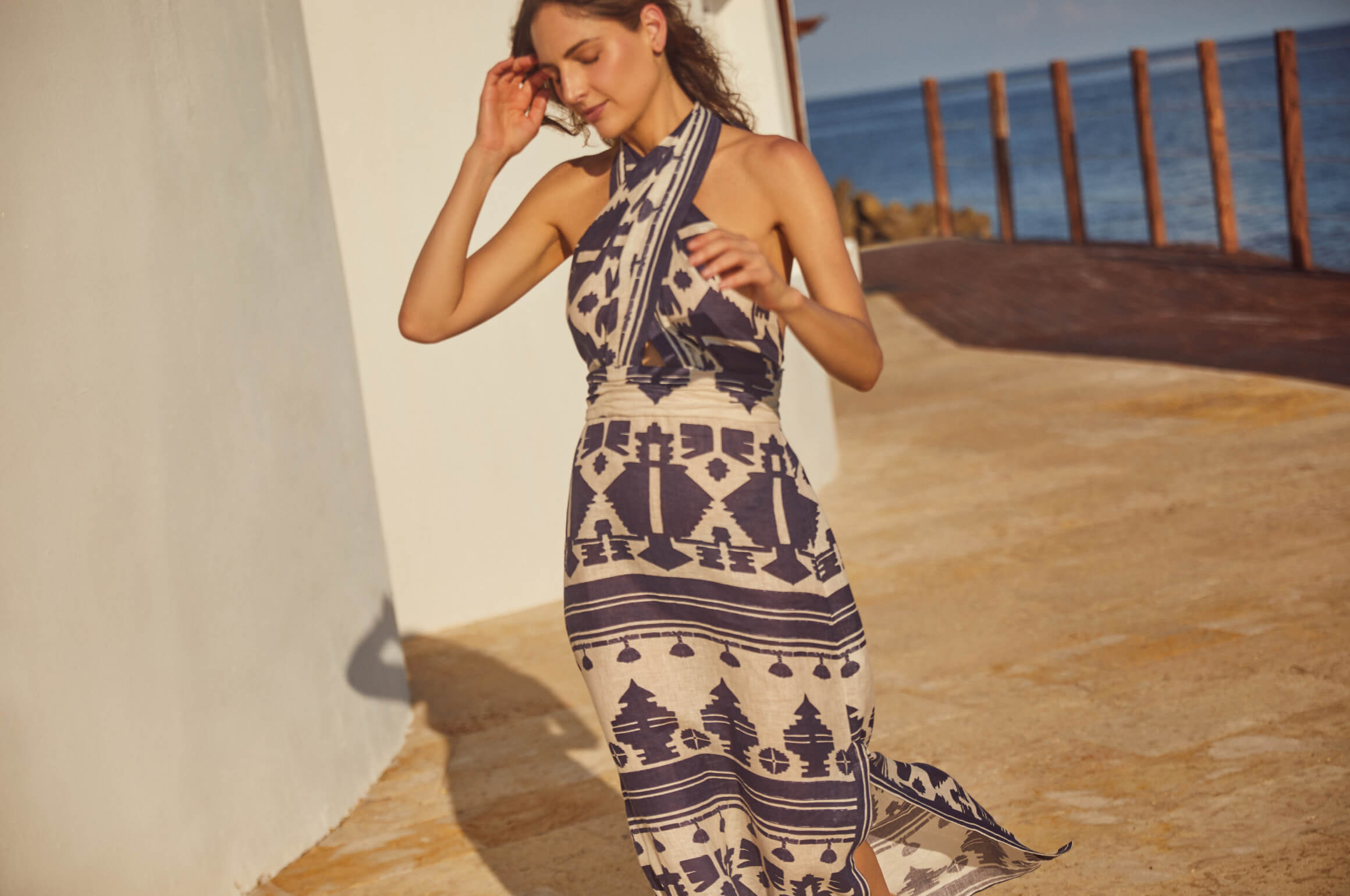This detailed photographic image captures a young white woman, likely in her 20s, standing outdoors during the daytime. She is wearing a long, flowy sundress that extends to her ankles with a left-side slit revealing her leg. The dress features cross straps over the shoulders, leaving them bare, and it is designed with a blue and beige tribal Aztec pattern, including stripes, bars, and plus signs or crosses. Her eyes are closed as she looks down, with her right hand resting on her forehead and her left arm extended upwards in front of her chest.

The scene is set against a backdrop of a white plaster wall to the left, a beige ground beneath her feet, and six wooden poles visible in the background to the upper right. Beyond the poles, a serene body of blue water stretches out under a clear blue sky. The overall composition features no text, focusing entirely on the serene and contemplative mood of the subject and her surroundings.